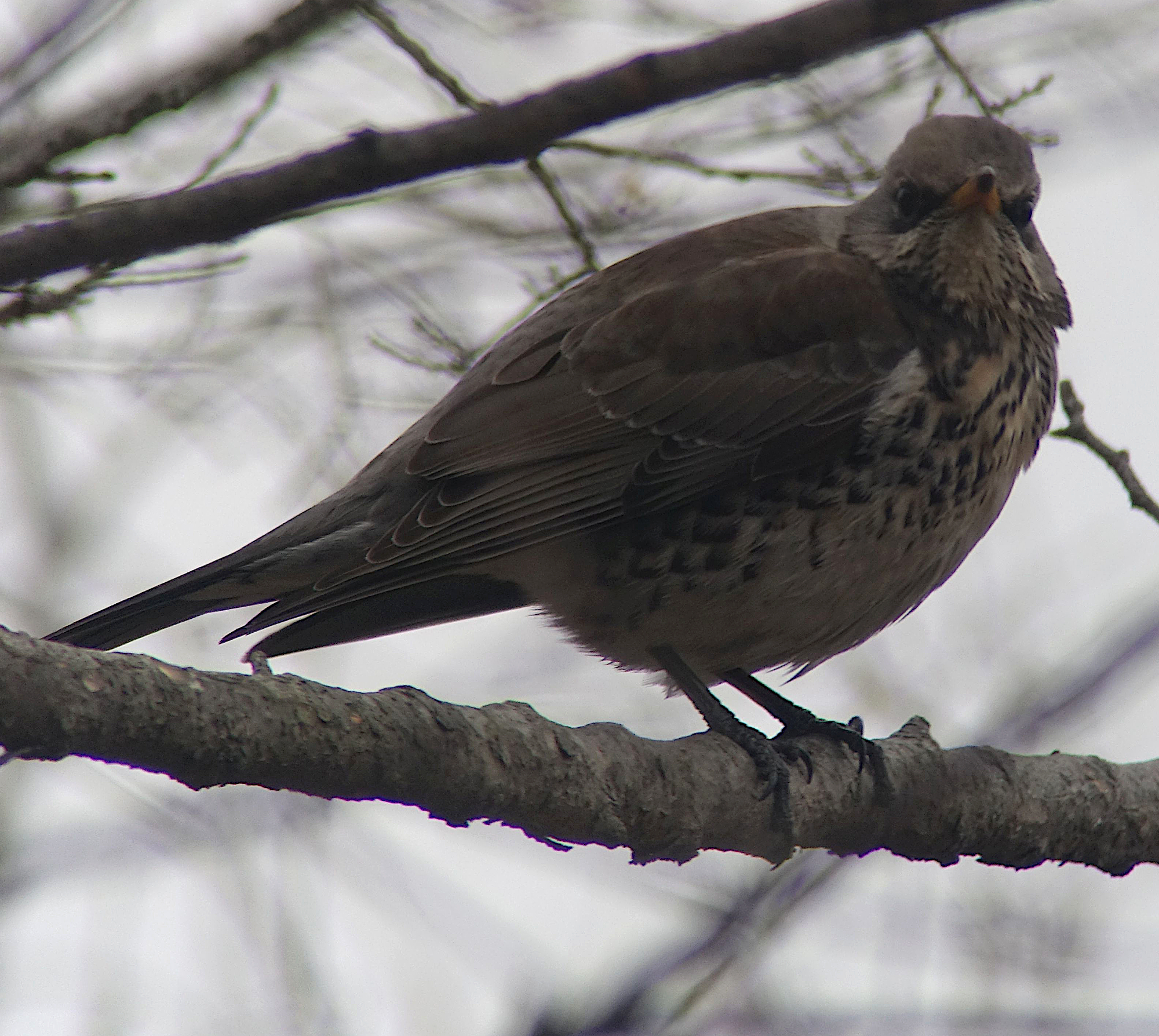This close-up square photograph captures an adorable, large brown bird with striking details. The bird, predominantly in various shades of brown and tan, is perched on a semi-thick branch, holding on tightly with its webbed feet, seemingly high in the trees under a muted sky, possibly suggesting early morning, early evening, or a cloudy day. Its big, dark eyes gaze directly at the camera while its short, orange beak adds a touch of contrast to its earthy palette. The bird's feathers are meticulously detailed, showcasing the intricate layering and texture. The background is blurred, ensuring the focus remains on this puffy, somewhat chunky bird, who appears to be watching something intently, capturing a moment of serene observation.